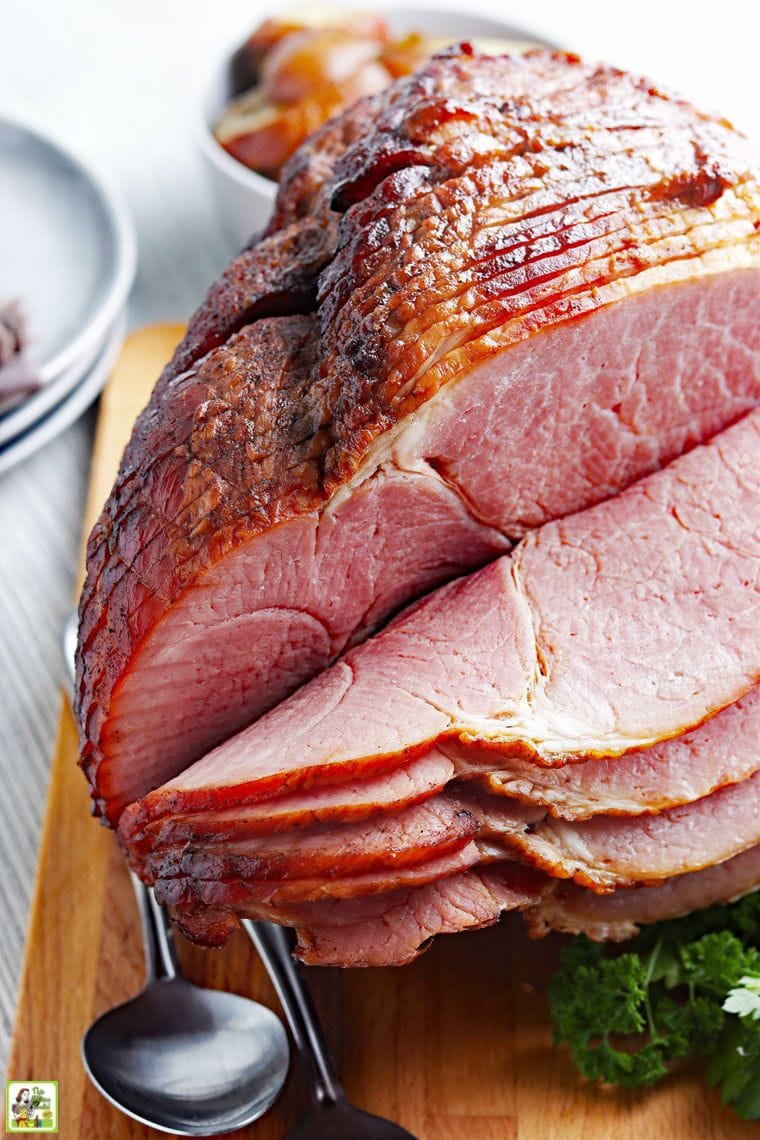The image features a meticulously sliced, spiral-cut ham displayed on a wooden cutting board set against a white background, likely a countertop. The ham, characterized by its enticing pink hue and decorated with golden-brown, braised, and possibly glazed spots, appears remarkably delicious. Thinly cut, the slices of ham curl and fold over one another in the foreground, creating a visually appealing presentation. Below the ham, a sprig of what seems to be kale adds a touch of green. The cutting board is also adorned with two metal spoons. In the background, slightly out of focus, there are three stacked plates and a dish that might contain stuffing. A very small watermark featuring a woman in a kitchen can be found in the bottom left-hand corner, but the main focus remains the enticing sliced ham laid out in succulent layers.